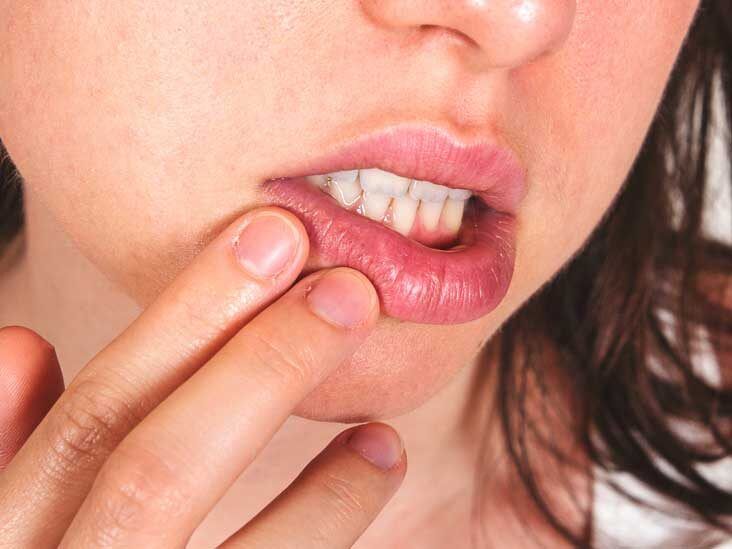This close-up, full-color photograph captures the lower portion of a young Caucasian woman's face, showcasing intricate details of her features and expressions. Her slightly open mouth reveals her immaculate, white teeth, while her lush, full, pink lips are gently pulled down by her fingers. The woman's skin is fair, and the bottom of her nose and her cheeks are visible. Her short-cropped nails, indicative of a nail-biter, hint at a possible sense of anxiety or discomfort, while her fingers touch her lips as if to reveal something, possibly suggesting dental pain or an attempt to draw attention to her teeth. Brown hair gently frames the right side of her face, cascading past her shoulder. She wears a white top, partially visible near her shoulder, further adding to the staged yet intimate feel of the photograph. The image's square format lacks a discernible background, focusing attention entirely on the detailed depiction of her facial expression and posture.